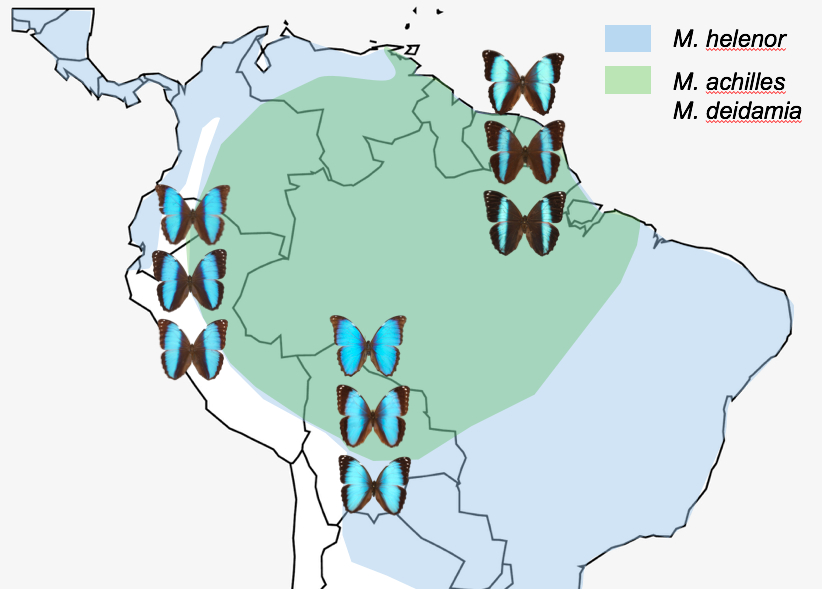The image depicts a detailed map showing the northernmost part of South America, specifically illustrating the distribution of three butterfly species: M. Hellenor, M. Achilles, and M. Deidamia. The map itself features a light gray background, with the continent outlined and segmented in white, light blue, and light green to indicate different butterfly habitats. The top right-hand corner includes a color key matching these species to the map's colors: light blue for M. Hellenor, green for M. Achilles, and another green variant for M. Deidamia. Overlaying the map, there are nine butterfly images—each rendered in black with turquoise blue details—stacked in groups of three. The butterflies follow this pattern: three in the top right, middle, and left-middle sections of the map. The detailed coloring and placement effectively highlight the geographic distribution of these species across the region.